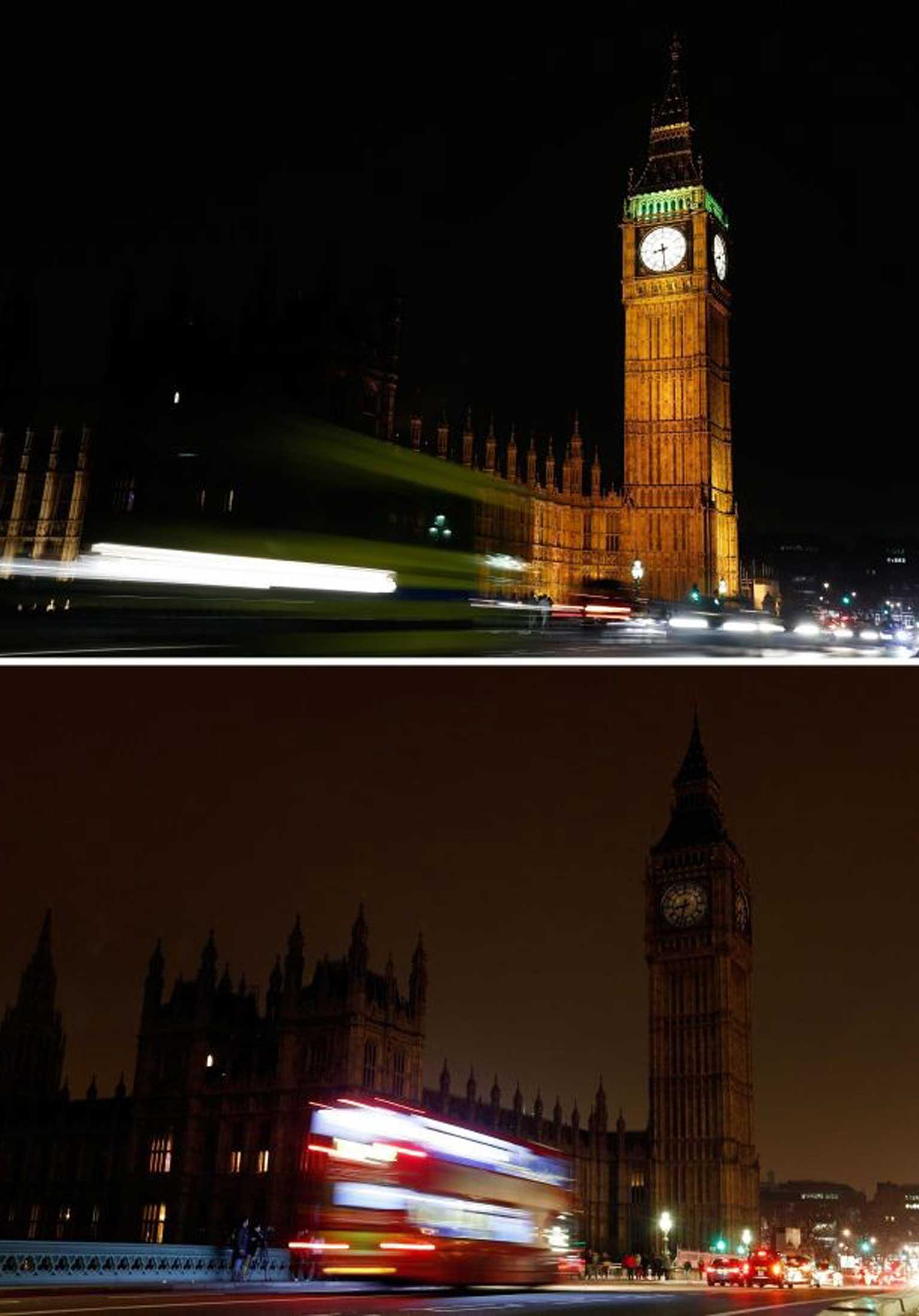This is a composite image featuring two stacked nighttime photographs of Big Ben, each capturing the scene at different times. The top photograph showcases Big Ben's iconic gothic architecture with its clock face lit up, displaying the time as 8:30, surrounded by a green illumination. The scene is vibrant with blurred lights from passing traffic, including a long white light streak on the left. The sky has a dark, murky tone typical of illuminated urban nights. 

In contrast, the bottom photograph presents Big Ben with its clock face not illuminated, suggesting a darker, perhaps later time of night. A double-decker bus, rendered into streaks of light from its motion, moves to the left, complementing the array of taillights from stationary traffic on the right. The pedestrian movement adds a dynamic, bustling street atmosphere. The overall scene emphasizes the difference in lighting and activity between the two times, capturing the perpetual motion of the city streets around this historic landmark.